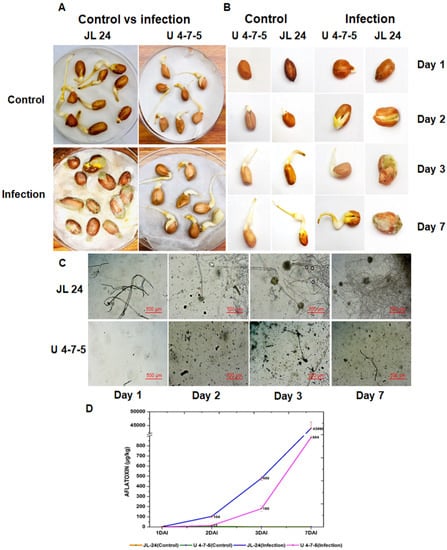The image is a detailed chart from an experiment involving beans, illustrated through multiple panels. The chart is divided into two main sections: the top section and the bottom section.

**Top Section:**
- **Left Side:** Represents Condition A with control versus infection.
- **Right Side:** Represents Condition B with control and infection.
- Both the left and right sides are organized horizontally to show the progression over days - day one, day two, day three, and day seven.
- The top row of images shows the control group, while the bottom row illustrates the infected beans. The images depict beans sprouting, clearly showing differences between the sprouting patterns in control and infected beans.

**Bottom Section:**
- Includes eight main panels, split into:
  - **Top Row:** Labeled CJL24, showing bean conditions over day one, day two, day three, and day seven.
  - **Bottom Row:** Labeled U4-7-5, displaying the same timeline progression.
- Each row compares how the identified bean variants perform under control and infected conditions.

**Additional Detail:**
- At the very bottom of the chart, there is a line graph, though the text details are too small to read. This graph features two lines: one blue line that ascends sharply and a purple line closely following but with a slight drop at the third data point. The lines likely represent different types of control and infection outcomes.

This structured visual representation offers a comprehensive view of how infection impacts bean sprouting over several days, with specific attention to different conditions and bean variants.